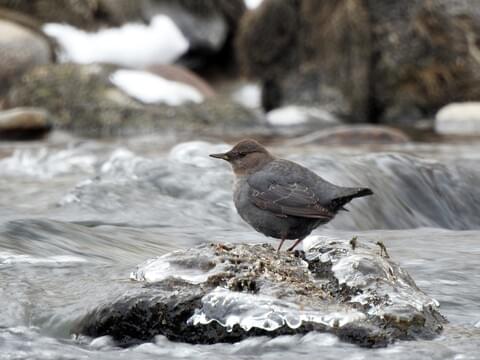This color photograph captures a stout, dark gray bird with a lighter brown head and shiny black eyes. The bird, distinguished by its circular shape and a pointy, light brown beak, stands on a rock in the middle of a swiftly moving stream. Its wings are tucked under, displaying a hint of brownish coloration, while its brown feet grip the ice-covered, gray rock.

Positioned in a side profile with its beak facing left and tail feathers to the right, the bird seems unfazed by the dynamic surroundings. The water splashes around the rock, creating rapid-like motions. In the background, a tiny waterfall cascades, adding white foam to the scene. The surrounding landscape comprises brown and gray rocks, many topped with patches of moss and snow, along with sparse grass. This serene yet powerful nature shot emphasizes the contrast between the static bird and the lively river backdrop.